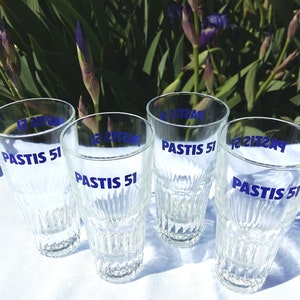This is a high-quality photograph featuring four tall, empty drinking glasses arranged on a table covered with a white tablecloth. Each glass, made of clear crystal, displays the text "Pastis 51" in dark blue or purple uppercase letters on both the front and back. The glasses are adorned with a prismatic crystal pattern around the edges, adding a textured, decorative element to an otherwise plain design. The table is set outdoors, and in the background, a multitude of purple flowers with green stems and leaves can be seen. The flowers are situated in a dimly lit area, providing a rich, contrasting backdrop that highlights the glasses in the foreground. The glasses cast subtle shadows on the white tablecloth, contributing to the overall serene and detailed composition of the image.